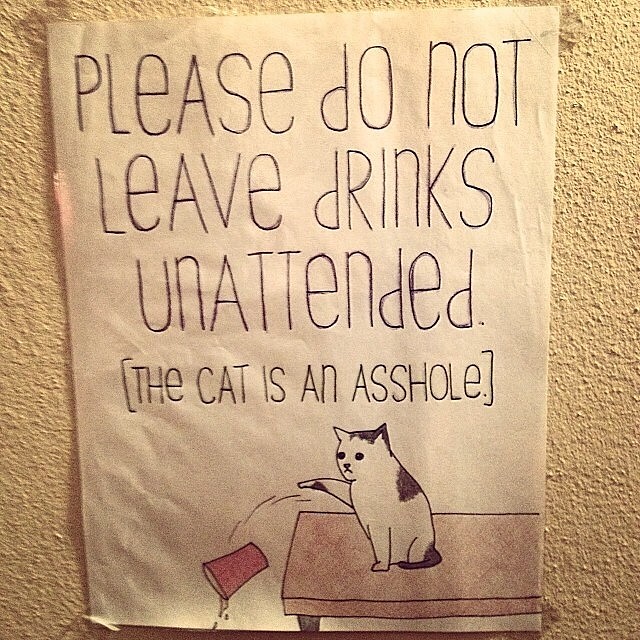In the image, a single object—a piece of artwork or sign—is prominently displayed, taped at all four corners against a textured, popcorn-like tan wall. The hand-drawn sign, positioned centrally, features the humorous text: "Please do not leave drinks unattended. (The cat is an asshole)." Below the text, an illustrated white cat adorned with black spots on its back, tail, and head, and one paw, is depicted swatting a red cup off a table, spilling its contents. This indoor scene, possibly within a kitchen, is colored in shades of tan, off-white, black, pink, and dark brown.